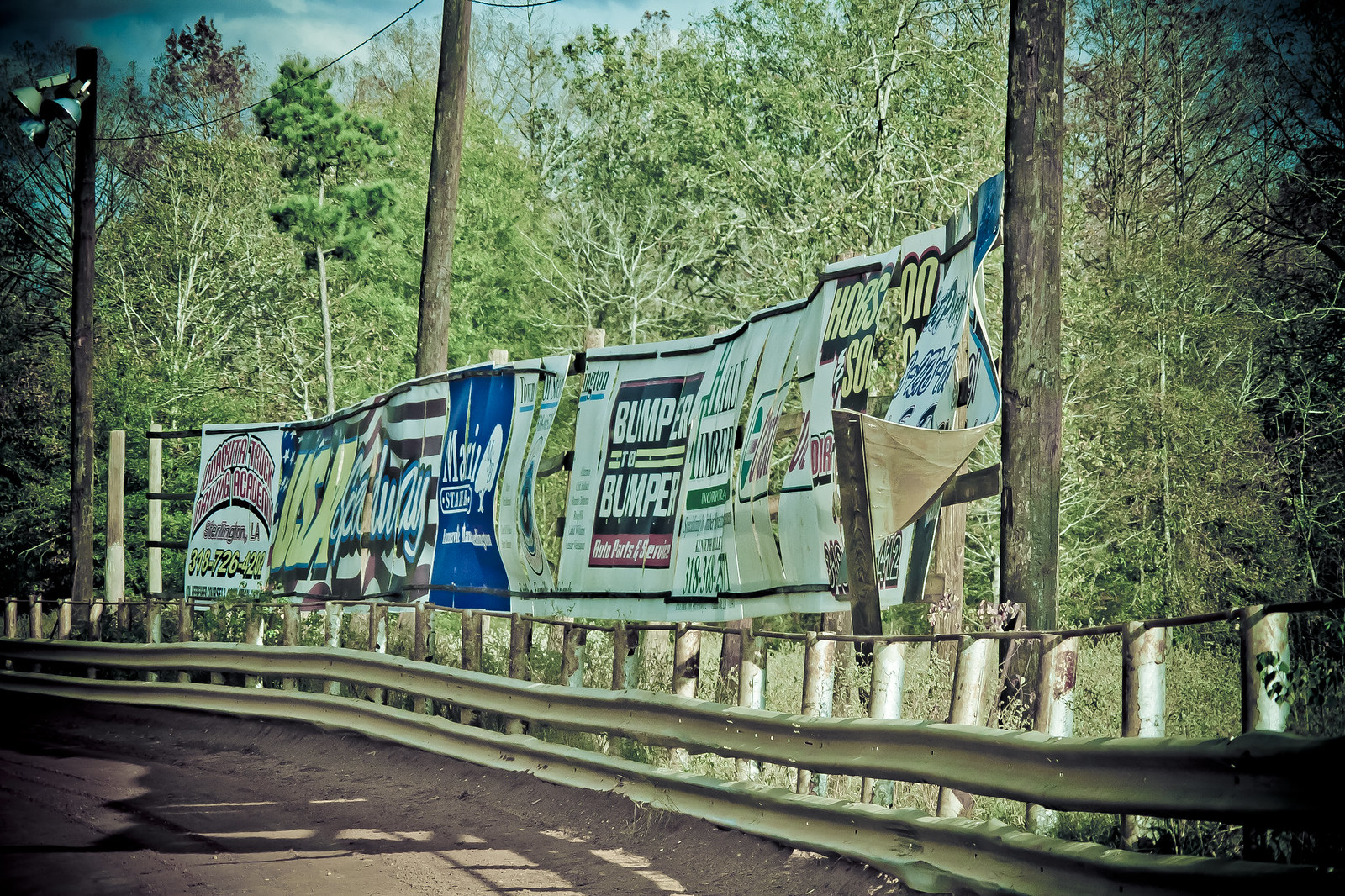This photograph, likely captured outdoors using a camera or a dashcam, depicts a curved rural road bordered by metal guardrails. The road starts from the bottom center of the image and curves quickly to the left, with a mix of gravel and dirt on the sides. Metal poles, showing signs of rust, support metal barricades designed to prevent vehicles from veering off the road. Utility poles draped with a single electrical wire and adorned with streetlights are visible, contributing to the scene's infrastructure. The background features a dense forest with large trees, some appearing unhealthy or dead, indicating a mix of seasons or forest health.

Above the guardrails, several canvas advertisements hang sporadically. Among the visible signs, one prominently displays "USA" with a flag, while another reads "bumper to bumper auto parts and service." The banners appear weathered with some torn and discolored, adding to the rustic, rural atmosphere of the scene. The sky above is mostly sunny with a few white clouds, casting a well-lit ambiance over the entire setting.